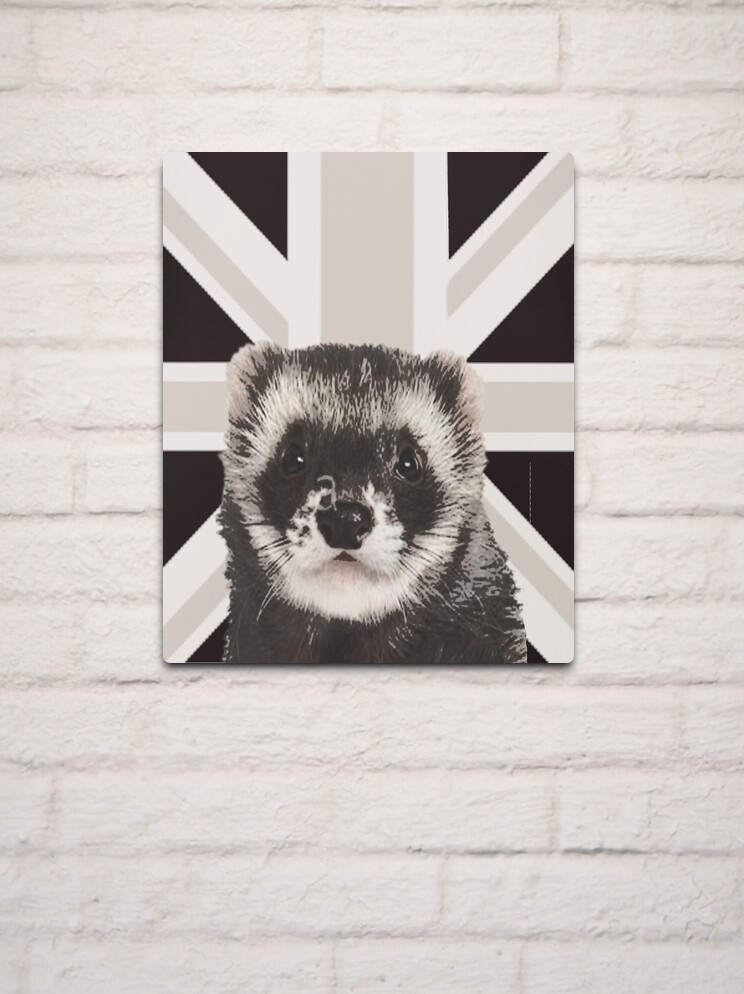A black-and-white photograph of a ferret is prominently displayed against a white painted brick wall. The ferret, facing directly forward with dark, penetrating eyes and a distinctive dark 'mask' around its eyes, contrasts sharply with the lighter fur surrounding this mask. The ferret's nose is black, complementing its whiskers, and its small round ears peek out from its dense fur. Behind the ferret is a Union Jack flag rendered entirely in black and white, enhancing the stark visual. The ferret image appears almost like a cutout, layered over the British flag, creating a striking, high-contrast artwork. This detailed, monochrome composition is mounted at the center of the white brick wall, creating a compelling focal point.